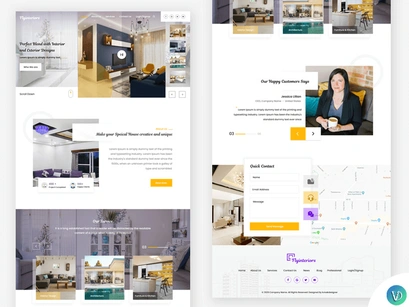The image consists of two website screenshots displayed in a side-by-side format. The left screenshot is unfortunately very small, making most of the text unreadable. However, its general layout can still be discerned. At the top of this left screenshot, there are two side-by-side images or slides. To the right of these slides is a narrow column. 

Below this section is a break that leads to a middle portion characterized by a plain white background. On the right side of this middle section is another image accompanied by some text. Following this is another distinct break that transitions into a new segment. This new segment features a background image with overlaid text, along with three smaller squares containing additional images positioned on top of the background.

The right screenshot appears to be a continuation of the page and is more detailed. It begins with another area that has a white background with an image and text overlay, mirroring the middle section of the left screenshot. At the bottom of the right screenshot, there is a map accompanied by some smaller text, likely providing additional information or navigation details.

Overall, the screenshots capture a website layout that incorporates a mix of images, text overlays, and background changes to create distinct sections throughout the page.